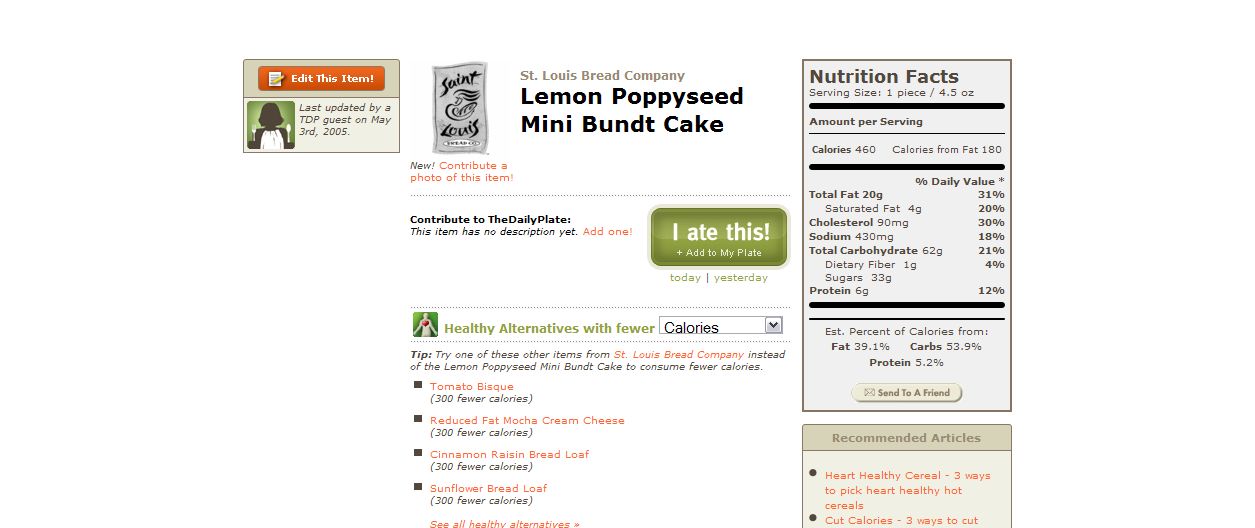**Image Caption:**

The image showcases a dated blog or forum page, characterized by an old-school website layout. In the top left-hand corner, there is a small box with a pencil icon labeled "Edit this item". Below it, there's an illustration of a woman prepared to eat, equipped with a spoon, fork, and bib. Adjacent to this, a note indicates the last update was made by a TDP guest on May 3rd, 2005.

Prominently in the center, the title "St. Louis Bread Company" is displayed alongside their logo. Below this, the featured item, "Lemon Poppy Seed Mini Bundt Cake," is mentioned with an invitation to "Contribute to the Daily Plate" as this item currently lacks a description. Users have the option to add this item to their plate by clicking "I ate this".

The webpage encourages choosing healthy alternatives with fewer calories, listing options such as Tomato Bisque and Cream Cheese. To the right, a detailed nutrition facts label for the Lemon Poppy Seed Mini Bundt Cake is provided, indicating a serving size of 4.5 ounces. The label includes information on calories, total fat, saturated fat, cholesterol, sodium, total carbohydrates, and dietary fiber.

Beneath the nutrition facts label, a section recommends related articles for further reading.